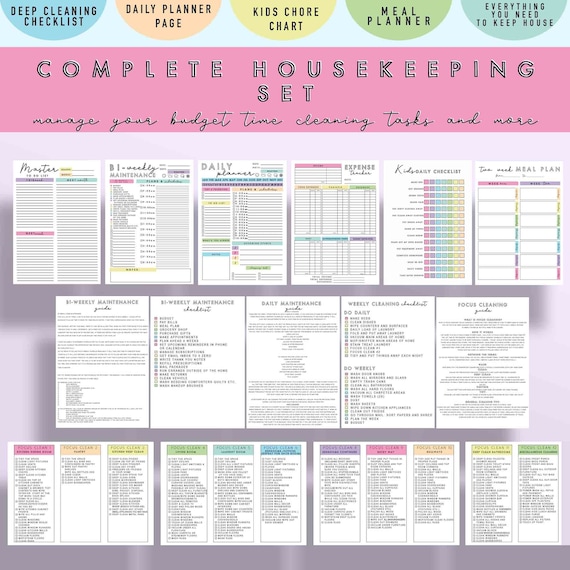The image is an infographic showcasing a "Complete Housekeeping Set" with the tagline "Manage Your Budget, Time, Cleaning, Tasks, and More." At the top, against a pink background, there are five color-coded half-circle tabs: "Deep Cleaning Specialist" (blue), "Daily Planner Page" (orange), "Kids' Chore Chart" (yellow), "Meal Planner" (green), and "Everything You Need to Keep House" (blue). The main content displays three rows of organizational slips. The first row contains six distinct tablets featuring meal plans and daily checklists. The middle row includes five sections of reading material, with content that’s difficult to discern due to the image being distant. The bottom row has four pre-written lists or checklists. This infographic appears to be a stock image promoting specialized planning pages for housekeeping tasks.